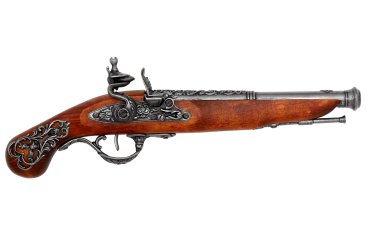The image depicts an antique, ornately designed flintlock pistol, possibly from the 17th to 19th centuries, set against a stark white background. The pistol features a single-shot mechanism characteristic of handguns from a few centuries ago, commonly associated with soldiers or pirates. The main body of the firearm is carved from a single piece of cherry-colored wood, giving it a rich, reddish hue. The metal components, including the barrel, hammer, trigger guard, and other firing mechanisms, appear to be silver or iron, though their age has darkened them to a nearly black patina. The intricate engravings on the metal parts and the distinctive shape of the trigger highlight its craftsmanship and historical significance. The gun, approximately 12 to 16 inches in length, showcases a blend of wood and metal, conveying both the artistry and functional design of its era.